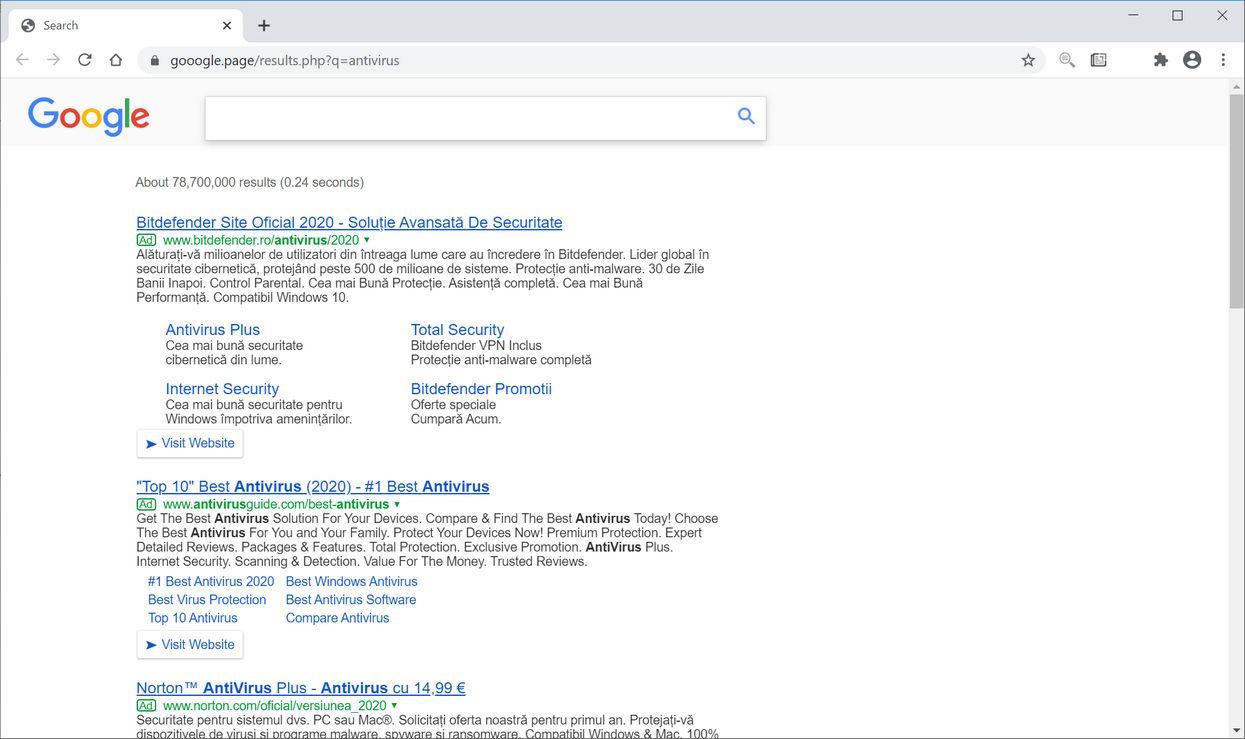The image is a screenshot of a Google search results page. The browser displays a single tab labeled "Search," featuring a small globe icon. The page has a clean, white background. In the upper left corner, the Google logo is prominently displayed, adjacent to a blank, white search bar. The search query appears to be related to antivirus software for computers. Four blue hyperlinks are visible in the search results. The top link reads "Bitdefender Site Official 2020" with additional text in a foreign language. The second link is titled "Top 10 Best Antiviruses 2020." The last visible link is "Norton Antivirus Plus Antivirus." The far-right corner of the page hosts an "Exit" button (an X), and a scroll bar is present on the extreme right side.